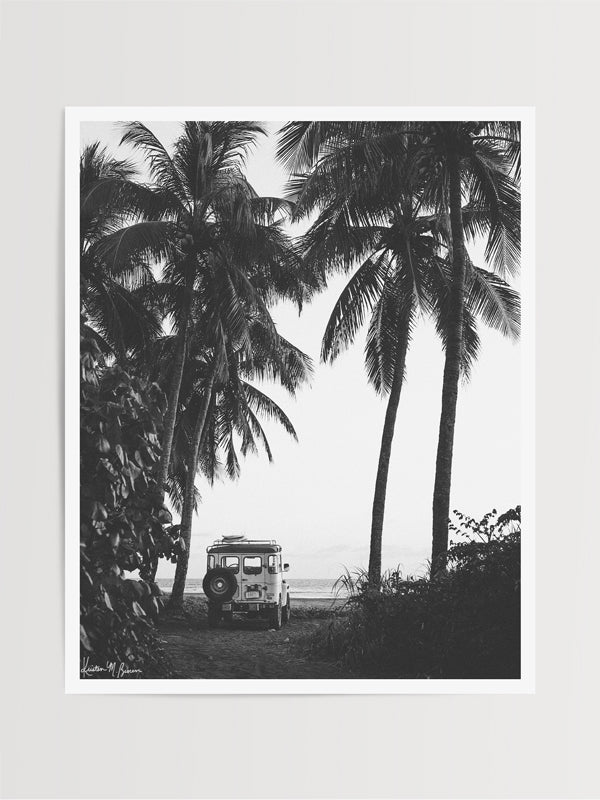This black and white photograph, which appears to be a scanned image, captures a serene beach scene featuring a small, white Jeep parked amidst a backdrop of tall, lush palm trees. The Jeep, viewed from the rear, conspicuously displays a tire mounted on its left side and has surfboards strapped to its roof. The scene is framed with four towering palm trees, two on each side of the vehicle, which dominate the image with their substantial height, standing roughly four to five times taller than the Jeep. Sparse bushes and shrubs can be seen scattered around the sandy ground, contributing to the natural setting. The ocean's horizon, with waves gently crashing in, stretches across the background, blending seamlessly with the grayscale sky. Notably, a signature, potentially reading "Kristen M. Russ," is inscribed in white in the bottom left corner of the photograph, which is set against a gray border. This visually captivating scene evokes a peaceful, nostalgic atmosphere.